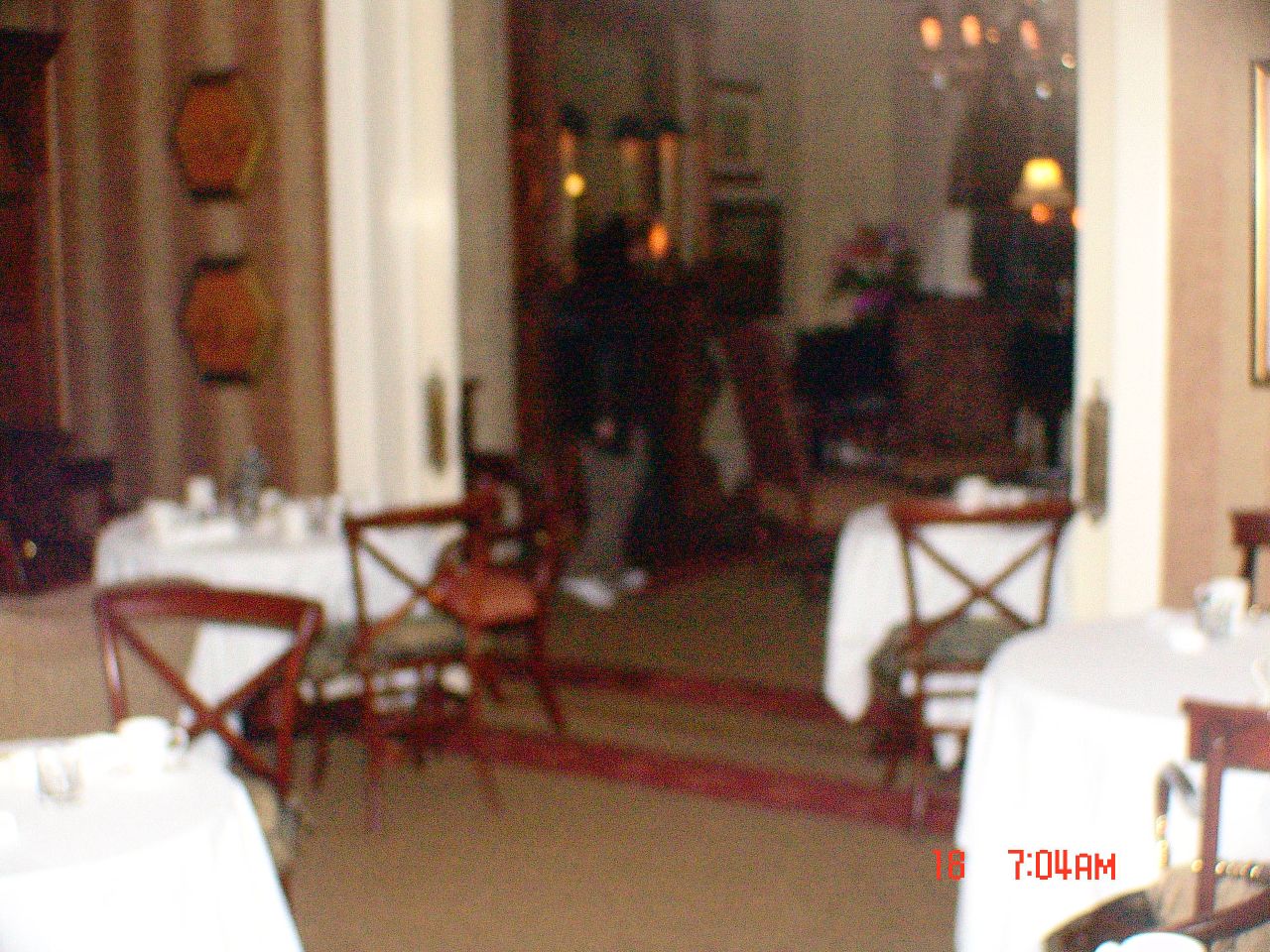The image depicts a blurred interior of what appears to be a quaint, non-chain restaurant that evokes the atmosphere of a bed and breakfast or a home business. The main dining area contains four small circular tables, each draped in pristine white tablecloths, linens, and napkins, and adorned with ceramic cups and possibly a silver centerpiece. The room has brown wooden chairs with gray seats, arranged around the tables, with at least one table being a two-seater. The floor is a brown carpet accented with red lines.

In the background, there's a woman standing near what seems to be a fireplace with a mirror above it. The wall's wallpaper alternates between light-colored and darker tan stripes. On the left side, two pictures are visible on the striped wallpaper, while to the right of the room's opening, there is a framed item on the wall, either in silver or gold.

In addition to the main room, another small room—a few steps up and accessible through open pocket doors—reveals additional dining furniture and a person partially visible in a dark jacket, brown pants, and white sneakers. A cabinet filled with unspecified items sits near another table. Timestamps in red text are visible on the bottom of the image, reading "18704 AM."